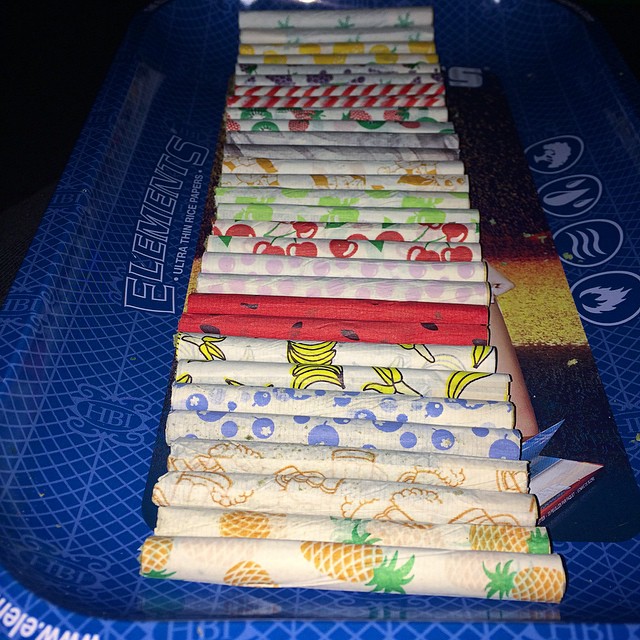This is a color photograph of numerous rolled joints, likely made from either marijuana or tobacco, neatly arranged within a blue rectangular tray that serves as a rolling station. The tray, identifiable by the text "elements ultra-thin rice papers" along one side, is designed specifically to hold these papers. The joints, wrapped in various styles of ultra-thin rice papers, are displayed prominently across the center third of the image, with many different vibrant patterns including pineapples, bananas, cherries, green apples, blue polka dots, pink bubbles, red cherries with green stems, and some with gold designs. The lower right corner of the image features the packaging for these rolling papers, while four circles on the tray's right side display symbols of tree, raindrops, squiggly lines, and a fire flame. The photograph is taken with the front in focus and the back blurry, giving the snapshot a depth effect as it captures the multitude of cylindrical rolls in various colorful designs.